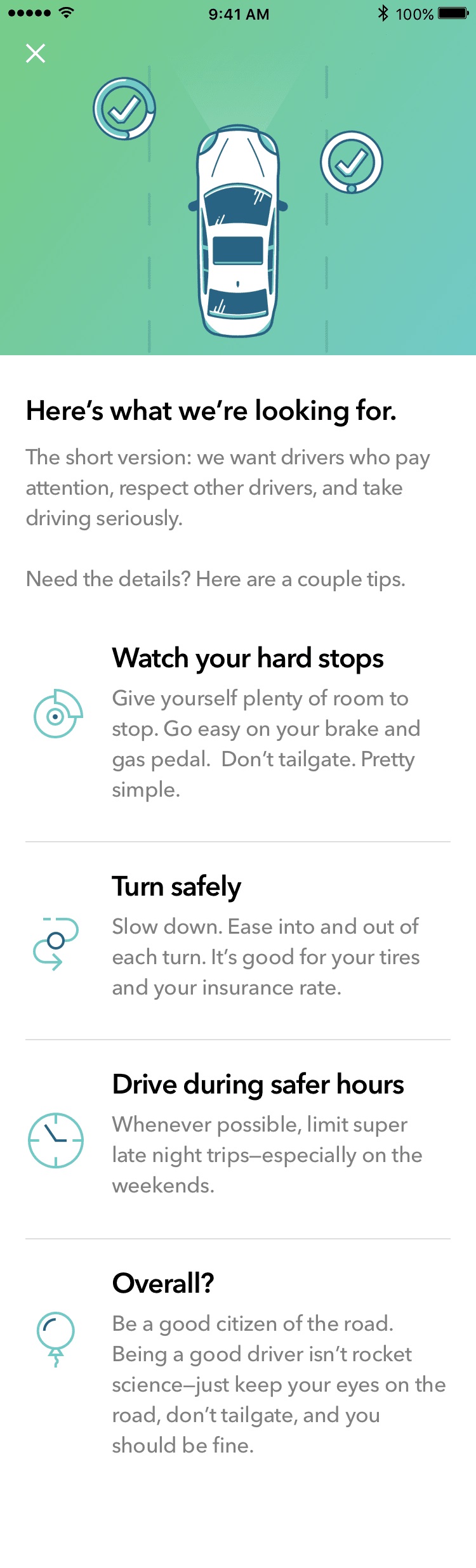The image displays a screenshot from a webpage featuring driving tips. The top section of the page is highlighted in green, showcasing an image of someone practicing driving. Adjacent to this image, there are several check marks indicating successful parking maneuvers. 

Directly below the green area, in a teal-colored section, there's text reading: "Here's what we're looking for. The short version. We want drivers who pay attention, respect other drivers, and take driving seriously." The section continues with more detailed advice: 

1. **Watch Your Hard Stops:** Give yourself plenty of room to stop. Go easy on your brake and gas pedal. Don't tailgate.
2. **Turn Safely:** Slow down, ease into and out of each turn. It's good for your tires and your insurance rates.
3. **Drive During Safer Hours:** Whenever possible, limit super late-night trips, especially on weekends.
4. **Overall** (followed by a question mark): Be a good citizen of the road. Being a good driver isn't rocket science. Just keep your eyes on the road, don't tailgate, and you should be fine.

The tips are written concisely and provide practical guidance for drivers to ensure safety and respect on the road.